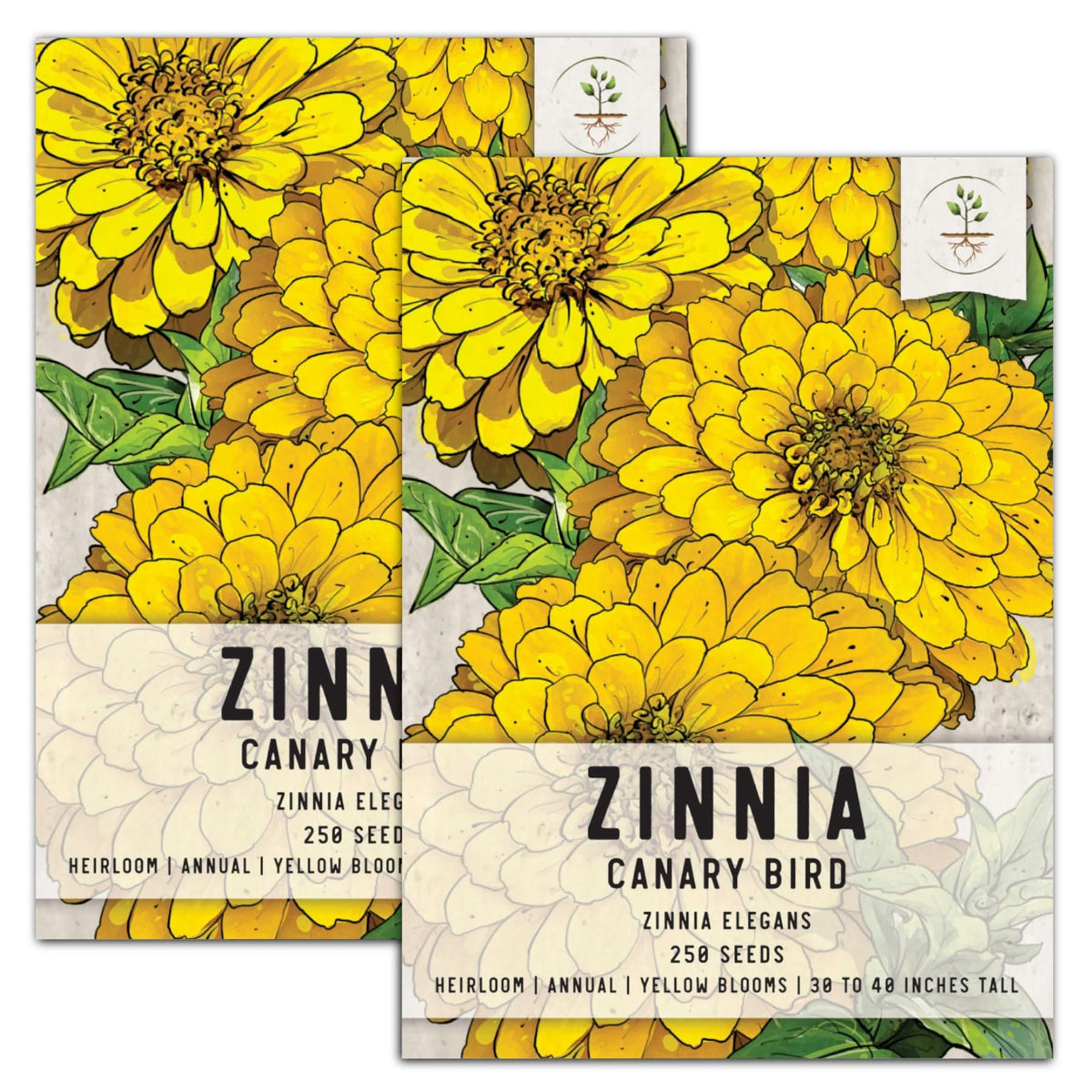The image depicts two identical seed packets for Zinnia flowers, with one packet slightly overlapping the other. These packets are labeled "Zinnia Canary Bird, Zinnia Elegans," and notable details include "250 seeds, heirloom, annual, yellow blooms, 30 to 40 inches tall." Each packet features an illustration of vibrant yellow Zinnia flowers, with two large blossoms prominently in the foreground and smaller ones behind, framed by the plant’s leaves. A distinctive emblem in the top right corner shows an outline of a plant with visible roots underground. The overall design of the packets targets retail display in store environments, highlighting the beauty and specific characteristics of these heirloom flowers.